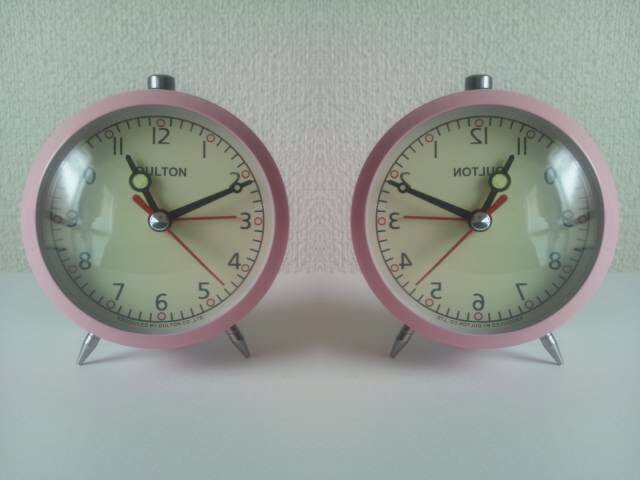This image showcases a pair of vintage-style alarm clocks set against a textured white wall and positioned on a pristine white mantle. Each clock features a pink rim with a white center, framing a dial face adorned with black hour markings from 1 through 12, each separated by minute markers. Two metal legs at the bottom angle outward from the 7 and 5 o'clock positions, giving the clocks a distinctive stance. The black hour and minute hands contrast against the face, complemented by a red second hand. The clocks are almost identical, but the one on the right displays its numbers as a mirror image of the one on the left, emphasizing their symmetrical arrangement. Both clocks have the brand "OULTON" inscribed at the top, and a silver metal piece on top, likely for setting the alarm.